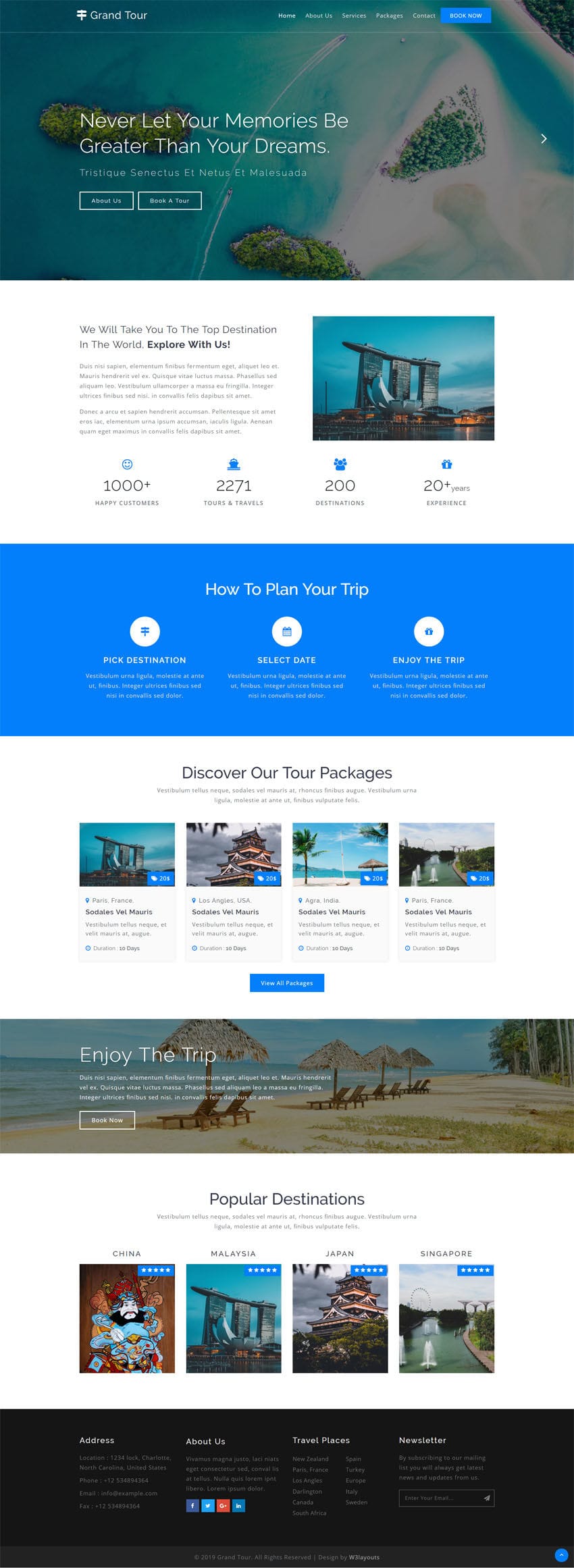The screenshot captures the homepage of a website, focusing on a visually striking beach scene viewed from above. At the top of the image, there are two tree-covered islands: one located at the top left and another at the bottom center. A narrow beach peninsula extends from the bottom-center island upwards to the right, while another beach can be seen in the top right corner, angled diagonally with a forest backdrop. Two boats navigate the waters between the islands on the left, leaving prominent white wakes behind them. The overall tone of the photograph is darkened, adding a moody atmosphere to the scene.

In the top-left corner of the frame, a white logo resembling a signpost icon is displayed, followed by the text "Grand Tour" in white. To the right, spaced evenly, are navigation links in smaller white text: "Home," "About Us," "Services," "Packages," and "Contact." Further right, there is a blue rectangle with white text that reads, "Book Now."

Prominently positioned in the center-left of the photograph is a large, inspirational message in white text: "Never let your memories be greater than your dreams." Below this, in smaller white text, is a Latin placeholder text: "Tristix and Tectus et Netus et Malaswada." On the far-right side of the image, a white arrow points to the right, located above two transparent buttons with thin white outlines and white text: "About Us" and "Book A Tour."

Beneath the photograph, the background shifts to white with a section titled, "We Will Take You to the Top Destination in the World," in dark gray text, followed by a bolded prompt: "Explore With Us." A light gray paragraph of text is situated below this on the left, providing additional information.